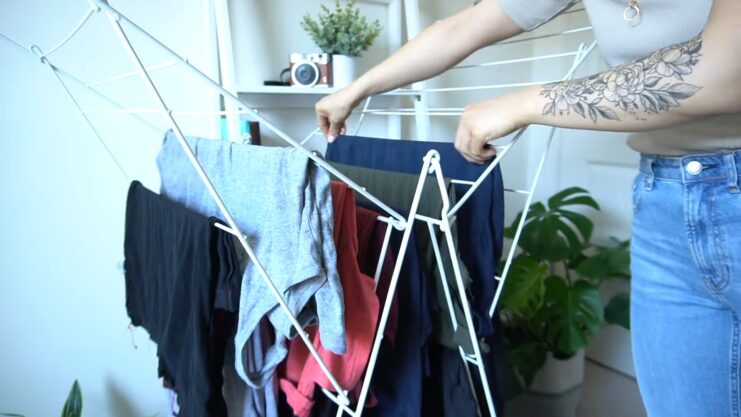In this image, a person is intently doing their laundry. Positioned to the right, the individual is a white Caucasian with a striking blue floral tattoo adorning their forearm. They are casually dressed in blue jeans and a gray short-sleeved top, accentuated by a gold chain partially visible with just the ring portion showing. 

An old-fashioned brown camera with a black lens sits at the top left, in front of a small white pot housing vibrant green branches. In the bottom right corner, another white square pot rests on the floor, also filled with greenery and displaying lush green leaves.

The backdrop is an off-white wall, free from shelving, but featuring a white plastic rack that supports the camera and the potted plant. A white door is visible on the right, and a white rack holds an array of clothes. From left to right, the clothes include a blue shirt, a gray top, a pink item, another blue piece, something green, and then yet another blue garment. This rack seems to be used for drying purposes. Adding to the modern aesthetic, the floor gleams with a shimmery gray finish.